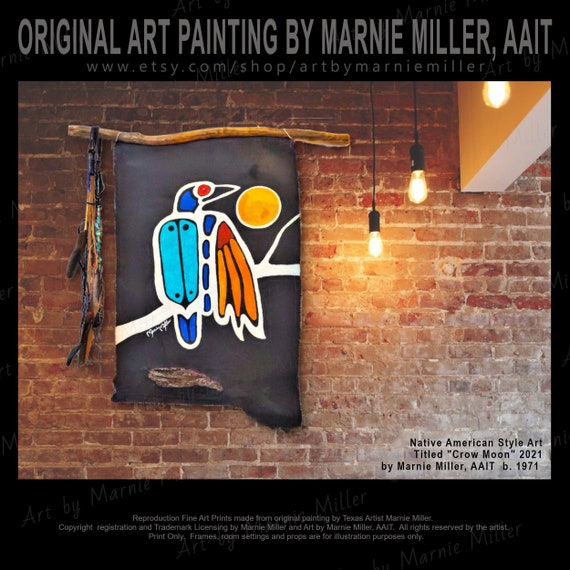The image depicts a weathered, distressed brick wall in what seems to be a stylish, artsy venue, either a club or a decorative art gallery. The modern architectural elements are highlighted by a beige support beam crossing the wall, which complements the rustic ambiance. Hanging from the ceiling are single-strand, amber-colored bulbs that illuminate the setting.

Prominently displayed on the brick wall is an art piece titled "Crow Moon 2021" by Marnie Miller. The artwork features a crow perched on a white branch, under a circular yellow moon. The crow's body showcases a palette of blue, red, and orange hues, creating a vibrant contrast against the dark backdrop of the flag-like hanging. The banner is affixed to a wooden stick, adorned with Native American decorations, such as feathers, at one end. Adding to the intricate detail, the flag has a small tear at the bottom, giving it a raw and authentic feel.

In the lower right corner of the piece, the name of the artist, "Marnie Miller," is prominently displayed. The surrounding area features hanging lamps with exposed, amber-colored bulbs on single strings, further enhancing the artistic and inviting atmosphere of the space.